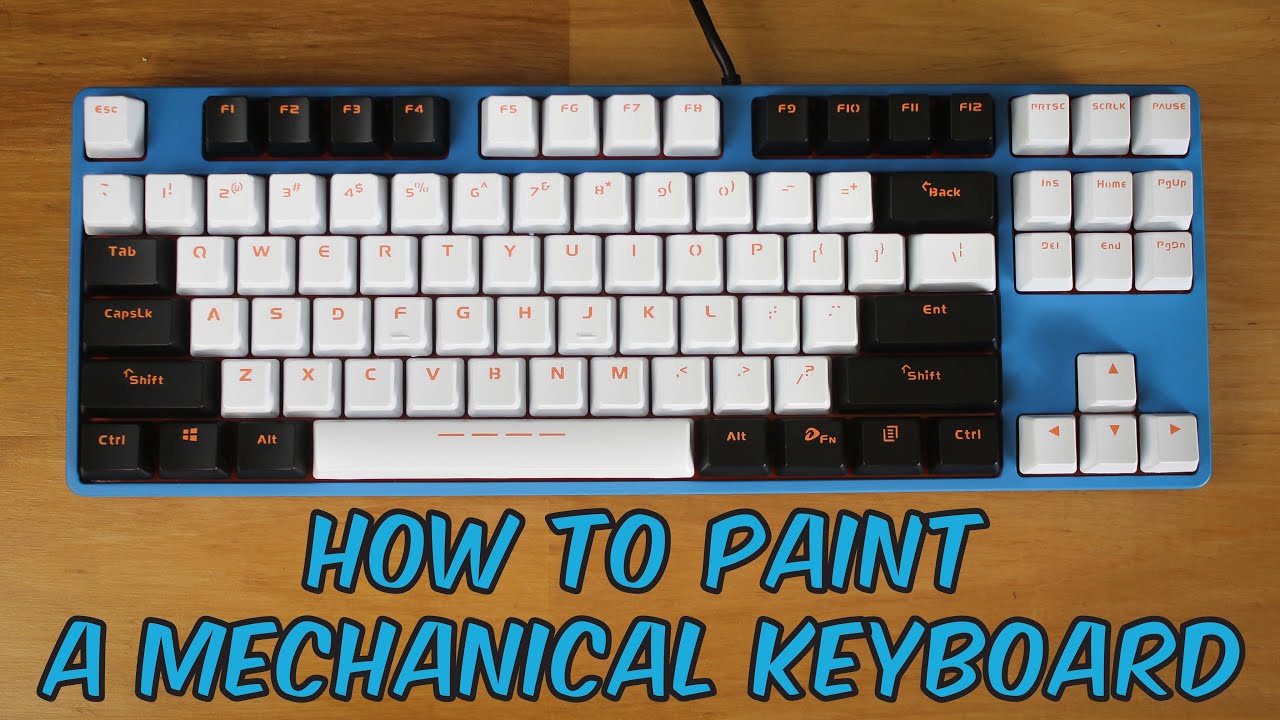An artistic advertisement for a custom-painted mechanical keyboard is showcased in this image. The keyboard, with predominantly white keys and select black keys for essential functions like Enter, Shift, Control, Alt, and Tab, sits gracefully on a rich brown wooden surface resembling a desk. Unique for its absence of number keys, the keyboard stands out with its sky-blue base, adding a refreshing burst of color. An electrical cord is connected to the back, trailing out of the frame. Below the keyboard, in bold light blue capital letters with a black border, the text reads, "HOW TO PAINT A MECHANICAL KEYBOARD," inviting viewers to explore the creative customization process.